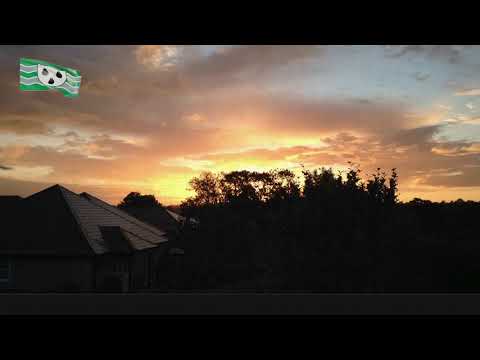The detailed image captures a sunset scene framed by black bars along the top and bottom. Dominating the top left corner is a green flag adorned with two grayish, zigzagging bars and a central white circle housing three black tear shapes, resembling droplets. Below this, to the left side, stand what appear to be three white pyramid-shaped tents or huts, their peaks extending upward. The right side of the image is heavily shaded by dark silhouettes of trees, obscuring part of the view. The sunset itself is a glowing yellow oval, embraced by dark brown clouds with a touch of blue sky visible in the top right corner. The overall atmosphere is dim with the sun's light struggling to penetrate the dense canopy and cloudy sky, creating a dramatic interplay of shadows and light.